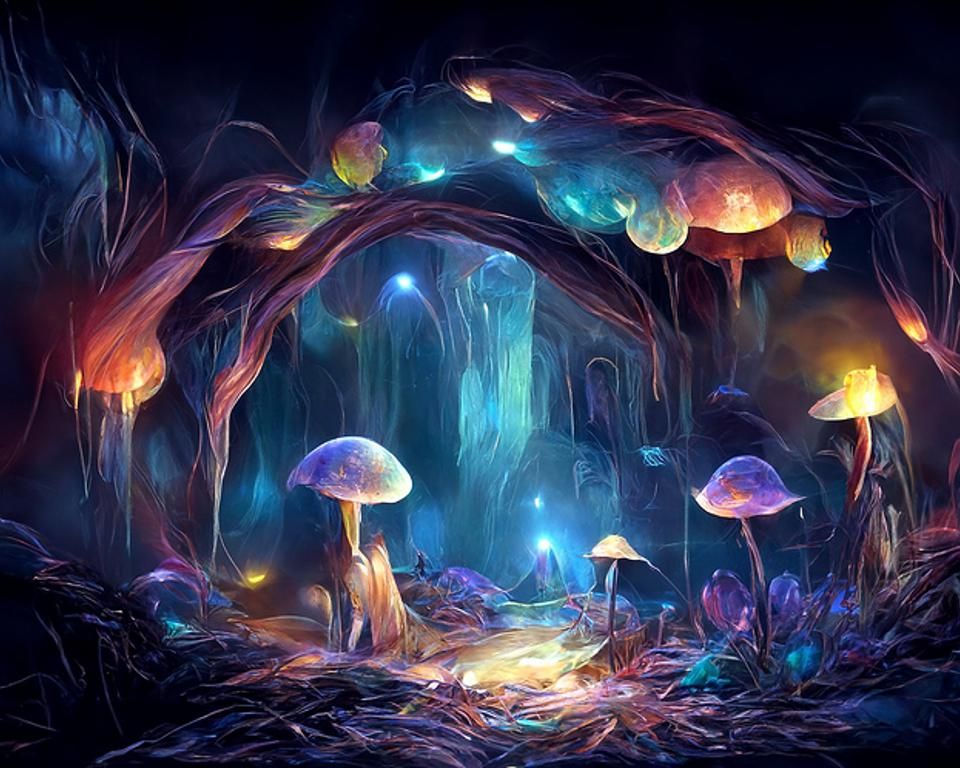This digital artwork captures the ethereal beauty of an underwater cave or a dreamy garden filled with bioluminescent jellyfish-like mushrooms and other glowing plant-like forms. The scene is saturated with vibrant hues, predominantly purples and blues, interspersed with reds, yellows, and greens. These colorful organisms appear to drape from the ceiling like chandeliers, casting an entrancing glow throughout the cavern. The ground is carpeted with intricate, marble-patterned mushrooms, resembling seaweed or dead plants, contributing to the mystical ambiance. Some clusters of mushrooms are neatly spaced, with a distinct arrangement noted on the left side and the right side of the image. The background is obscure and impenetrable, adding an air of mystery to this illuminated cavern. There are no discernible figures or text, enhancing the focus on the surreal botanical and marine elements. The entire scene conjures a fairy-tale world where the forest floor and underwater realms converge in a spectacular display of light and color.